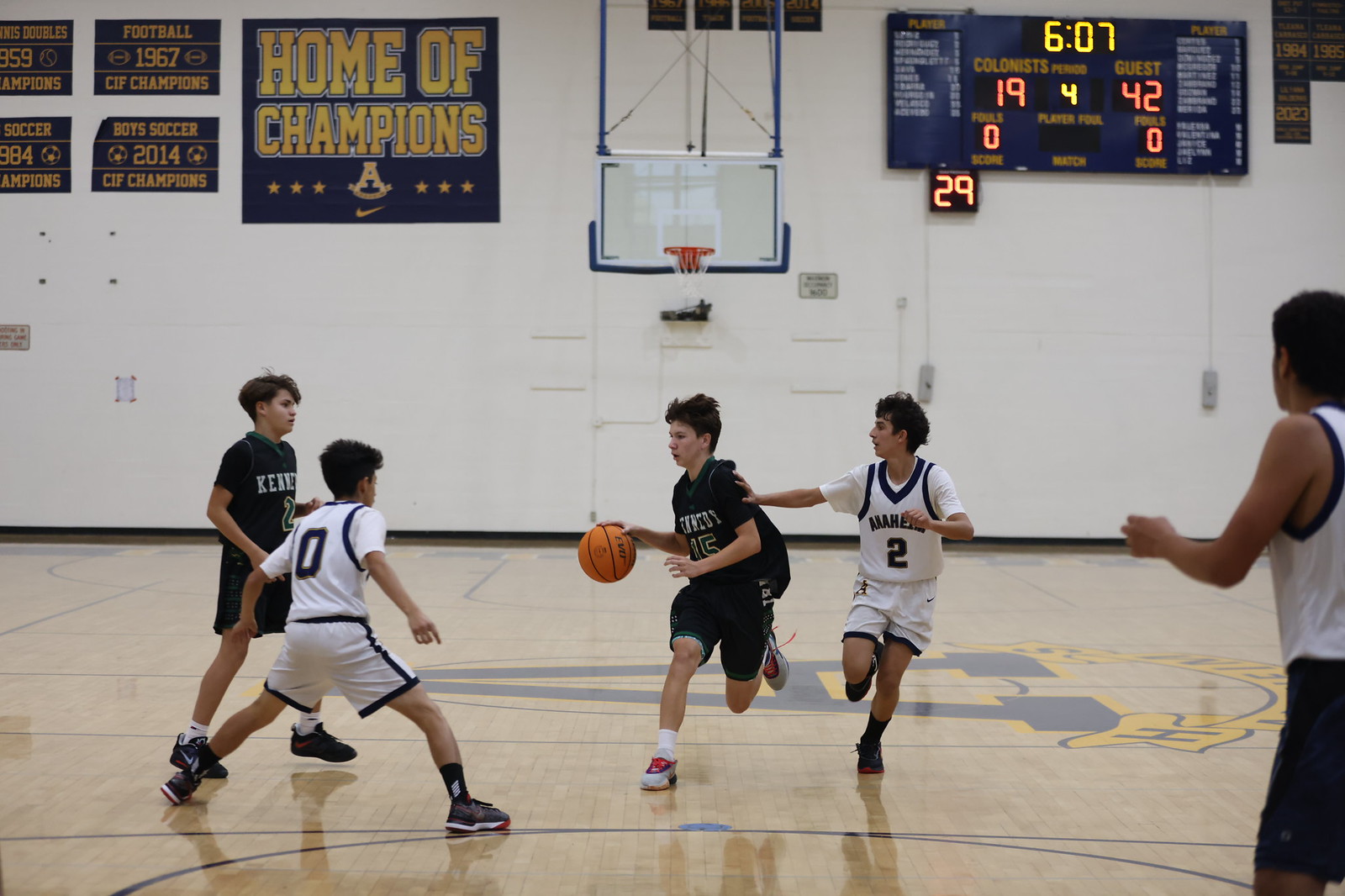The photograph captures an intense middle school basketball game taking place in a gymnasium with white walls and a wooden floor. The gym has a prominent black banner with bold yellow letters proclaiming "Home of the Champions". The dark blue scoreboard, showing 6 minutes and 7 seconds left in the fourth quarter, indicates the guest team leading with a score of 42 to 19. On the court, two teams of young boys between the ages of 9 and 13 are actively engaged. One team sports white jerseys and shorts with black piping along the edges, while the opposing team wears dark-colored outfits, with some descriptions noting them as dark green tops with black shorts featuring green bands. A player from the dark-colored team is captured mid-action, running and dribbling the ball. Behind the players, a basketball hoop hangs from the ceiling, contributing to the dynamic atmosphere of the game.